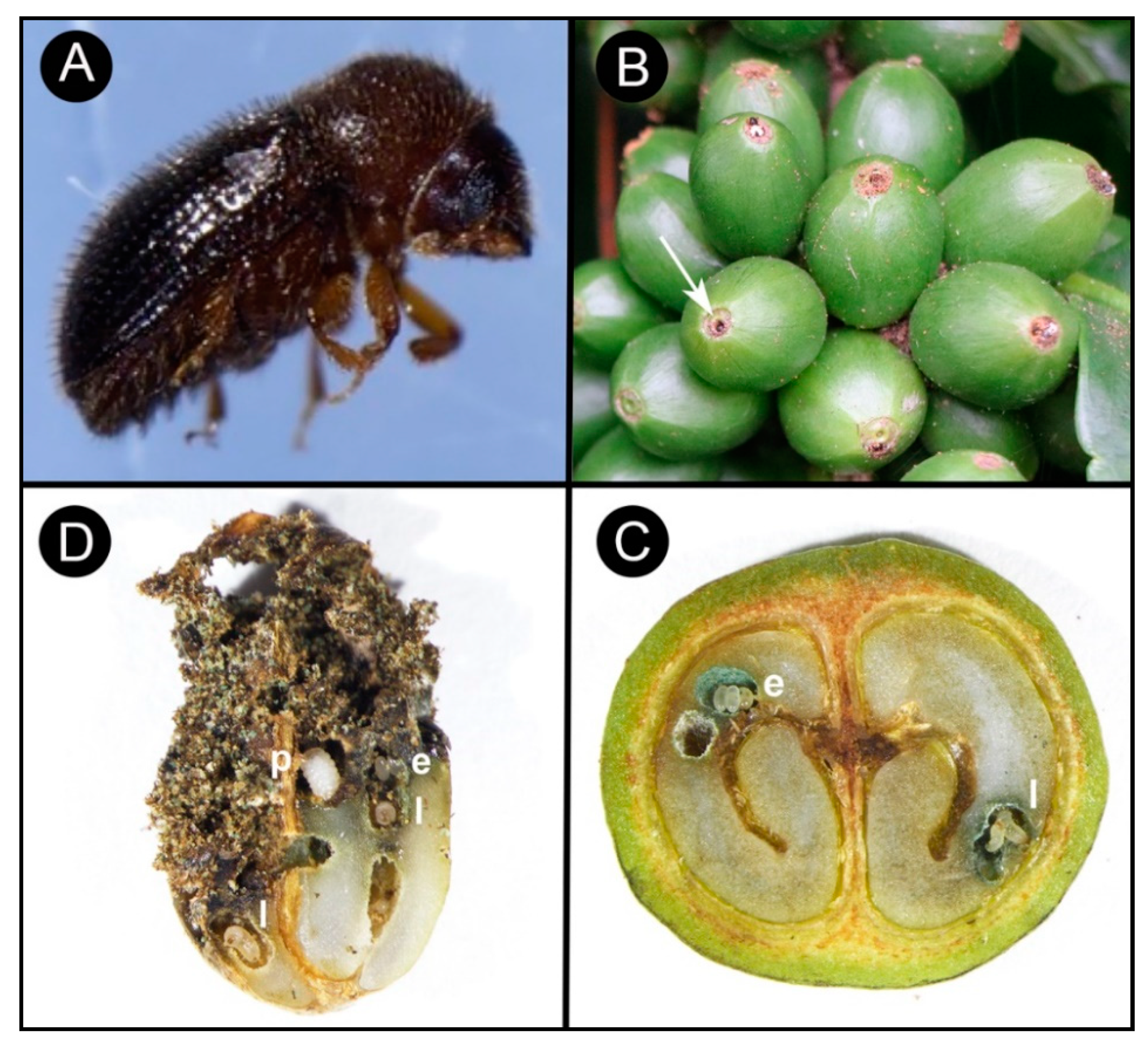This composite scientific panel depicts the life cycle of an insect, divided into four labeled sections: A, B, C, and D. Panel A shows a close-up of a full-grown, fuzzy brown insect, possibly resembling a bee, against a blue background. Panel B highlights a cluster of small green berries, with an arrow pointing to an opening on one berry. Panel C provides a cross-section of a berry illustrating sub-diagrams labeled E and I, displaying cavities within the fruit containing insect larvae. Lastly, Panel D showcases either eggs or more larvae consuming additional portions of the fruit, with locations labeled P, E, and I marking specific areas within the diagram. The detailed arrangement suggests an intricate look into the insect’s developmental stages within its vegetal host.